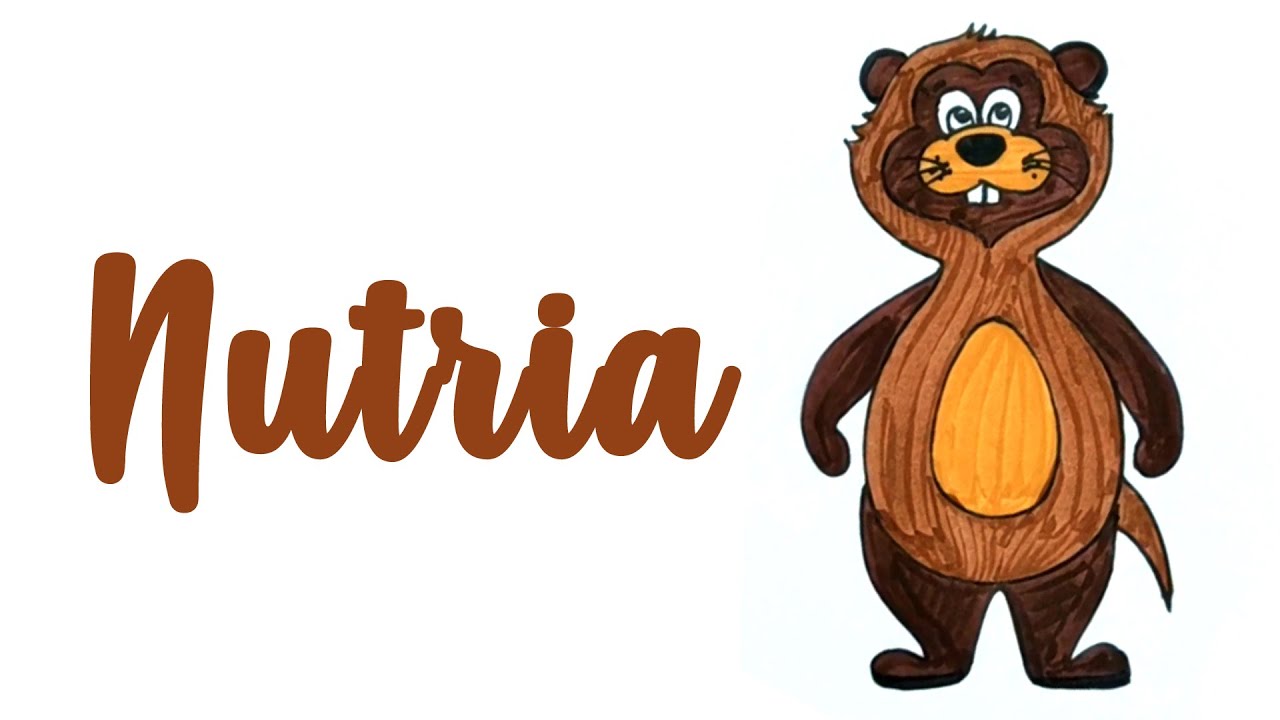On a crisp white background, a charming little beaver takes center stage, showcasing his endearing features. His face, a rich dark brown, contrasts beautifully with the lighter brown fur encircling his nose, which is a striking black. Prominent front and center are his two large, white teeth, nestled below his big, expressive eyes that gaze forward with a hint of curiosity and playfulness. Perched atop his head are his small, rounded ears that add to his adorable charm.

The beaver’s midsection is adorned with lighter brown fur, forming an almond-shaped patch of yellowish-brown right around his belly, distinctly standing out from the rest of his darker brown body. To his side, a prominent sign reads "Nutria," identifying this delightful creature. His overall demeanor exudes happiness, with his cheerful eyes looking upward and his little arms resting casually by his sides. This detailed depiction captures the essence of a joyous and undeniably cute beaver.